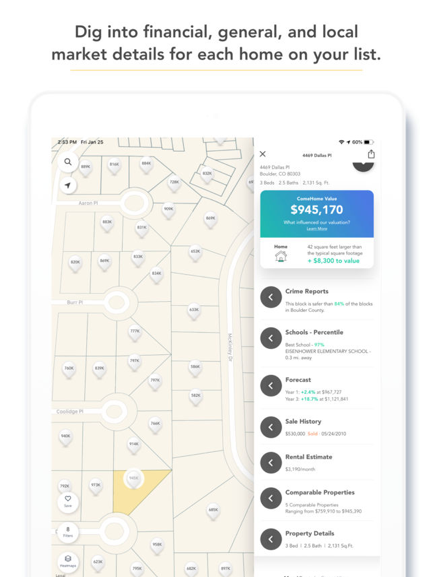**Detailed Caption:**

This image is a screenshot of a real estate application, likely accessed on a tablet or smartphone, as indicated by the visible time, battery, and service indicators at the top of the screen. The application appears to focus on providing comprehensive details about homes, including financial, general, and local market information.

At the top of the interface, a header reads: "Dig into financial, general, and local market details for each home on your list." Below this, the main content is divided into two sections. On the left side, there's a grid depicting plots of land, each representing a home. The grid itself is a beige color, with one triangular plot highlighted in a more pronounced yellow color, indicating it has been selected. 

To the right of the grid, information about the selected home is displayed. Although the text at the top of this section is quite small and blurred, making it difficult to discern, it includes an address in Boulder, Colorado. This might be indicative of the property's location. Below the address, the application's interface shows a property value of $945,170. Further down, additional statistics concerning the selected home are present but are also blurry and hard to read. The overall layout suggests a detailed and user-friendly interface designed to help users explore various aspects of real estate properties.